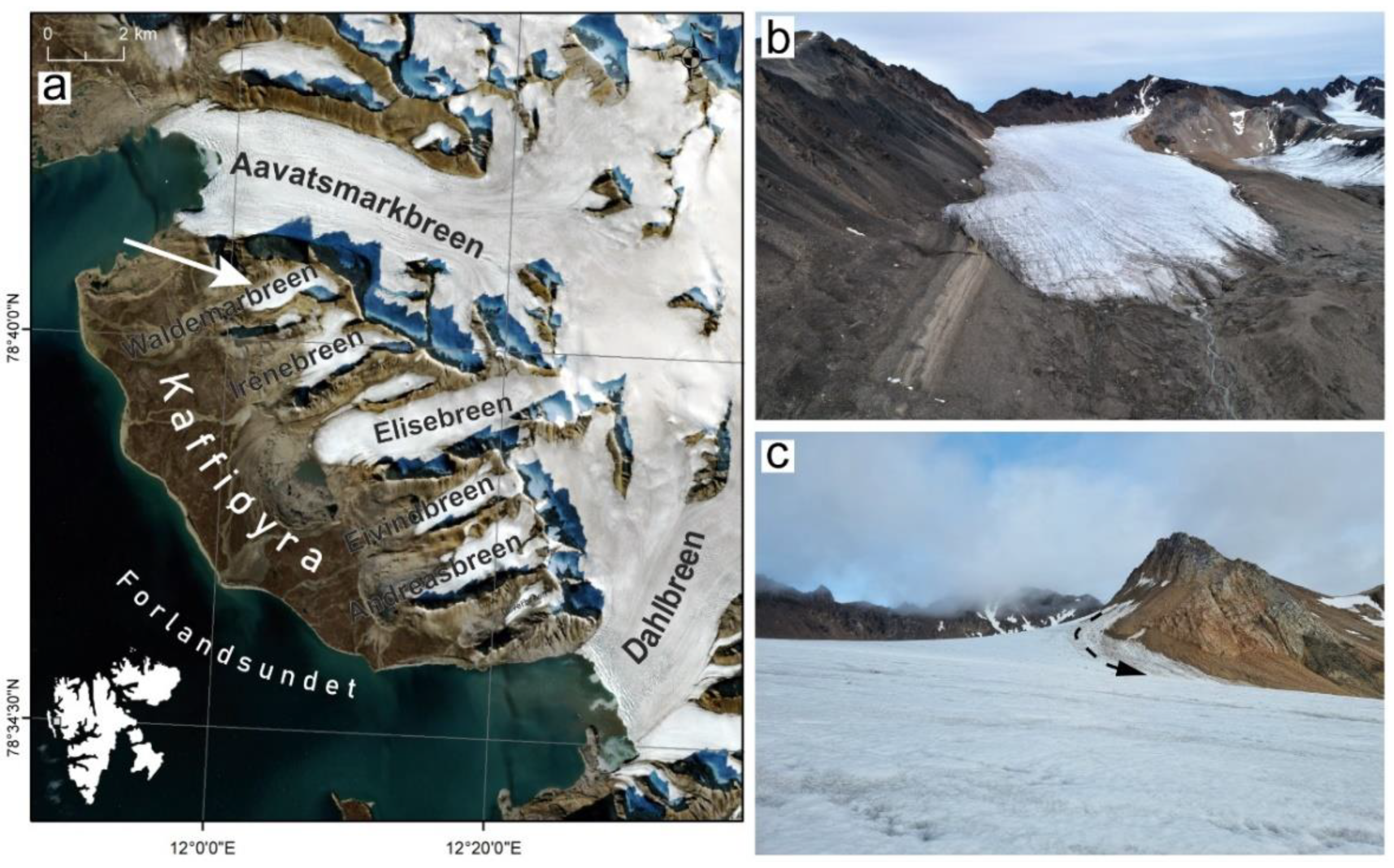The image is divided into three labeled sections: A, B, and C. Image A, located on the left, is an aerial illustration map of the Alaskan wilderness, showcasing a rugged terrain with glaciers, snow-covered areas, and dark brown land features. This map includes several place names written in what appears to be a Scandinavian language, such as "Avads Marks Breen," "Walden Vern Breen," "Lease Em Breen," "Kafurra," "Forland Sundet," and "Daw Green." The map is detailed with geographic indicators like contours and possibly elevation markers marked with numbers such as 1200 and the letter E. 

To the right, images B and C are realistic photographs capturing the Alaskan wilderness. Image B features a glacier, its talus extending down into soft dirt with a landscape of snow and low clouds in the background. Image C, on the other hand, offers a perspective from on top of the glacier, looking up towards rugged snow-capped mountain peaks partially obscured by low-hanging clouds, set against a blue sky. Together, these images provide a comprehensive view of the stunning and cold Alaskan environment.